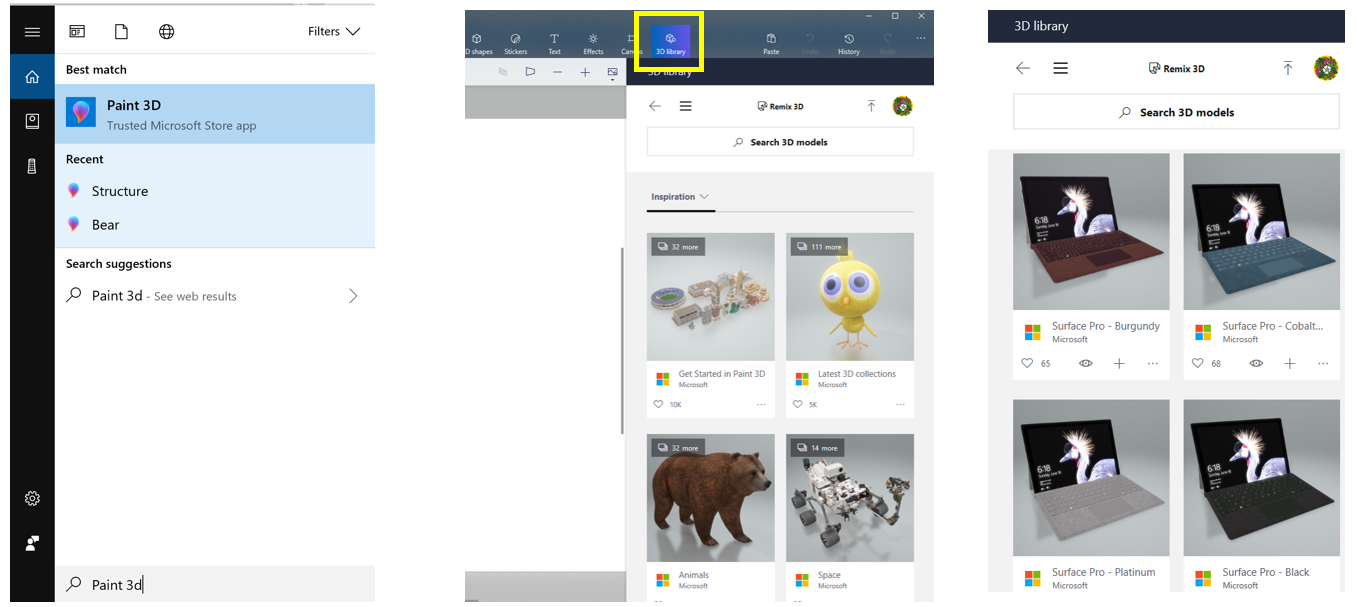**Detailed Caption:**

In a series of three screenshots displaying the Paint 3D application, the first screenshot on the left showcases the user accessing the Windows start menu. They've typed "Paint 3D" into the search bar, and the application is highlighted as the best match. Underneath, recent searches include "structure bare," and search suggestions indicate "Paint 3D" along with options to see web results.

The middle screenshot provides a glimpse into the Paint 3D app in action, featuring four notable 3D models: an upper right yellow duckling, a bottom right robotic car, a bottom left brown bear, and an upper left depiction of a football stadium accompanied by smaller buildings. Centrally, a yellow box highlights a specific tab in the interface.

The final screenshot on the right focuses on the 3D library section within Paint 3D. The upper left corner displays the "3D library" label, with "Remix 3D" in the middle, and a search bar prompting "search 3D models." Below, four laptops are depicted, each in a different color: maroon red (upper left), blue (upper right), black (bottom right), and white-gray (bottom left).